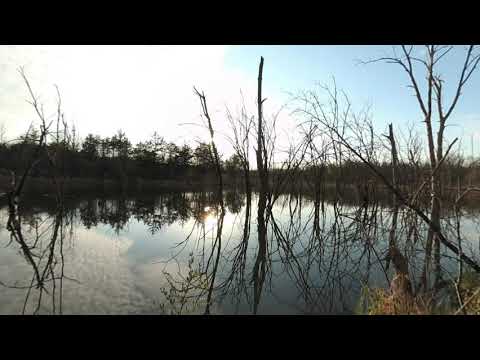The image captures a serene, smooth, gray-toned body of water at its center, flanked by dead, leafless trees and brown sticks that resemble lifeless bushes. A single weed emerges from the water just left of center at the bottom. On the left side, white moss carpets the water’s surface. Reflecting the contrasting vitality of nature, the left background showcases green, leafy trees, transitioning to bare, dead trees as you move right. The sky above mirrors this gradient, starting as a grayish tone on the left that fades into a light blue on the right. A notable light source, possibly the sun, is visible slightly left of center near the horizon, its reflection clearer in the water below. The entire scene is framed by black strips at the top and bottom of the image, adding a striking border to this evocative picture of a tranquil, yet starkly divided, natural landscape.